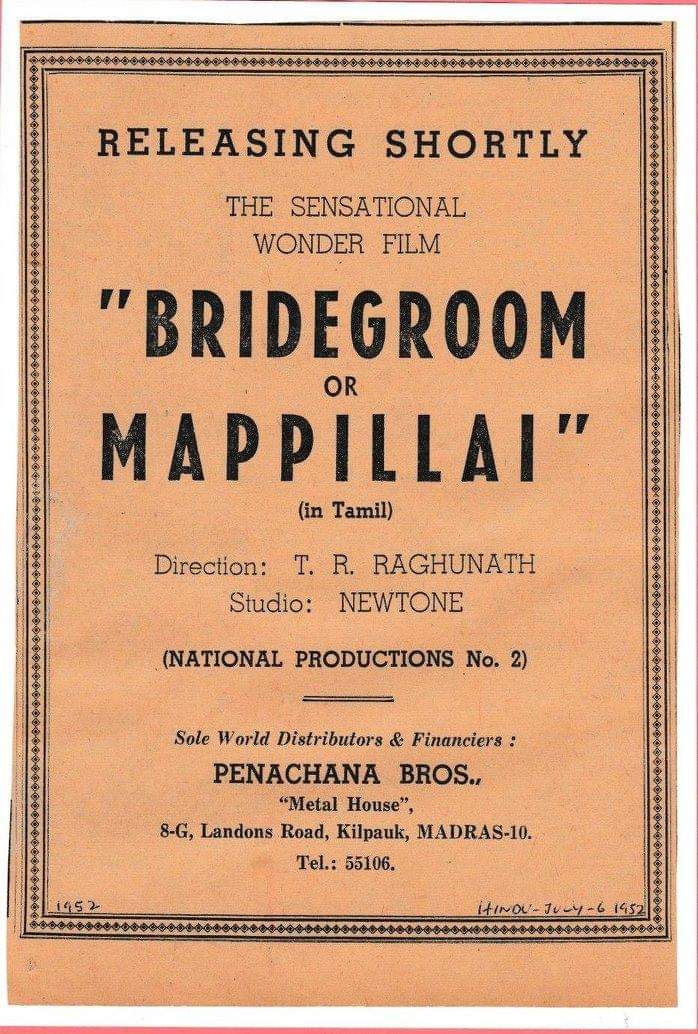This portrait rectangular image advertises a film and appears as a scanned sheet of old, orange-colored paper with a decayed, worn aesthetic reminiscent of old documents. The background is a peach or salmon hue, framed by a decorative geometric design of triangles or diamond shapes encircling the entire image. Layered over this ornate border, the black printed text stands out clearly against the faded backdrop.

At the very top in large, all-caps black letters, it announces "RELEASING SHORTLY." Just below, it describes the film as "the sensational wonder film" followed by the title in large quotation marks: "BRIDEGROOM or MAPPILAI". Beneath the title, in smaller parentheses, it clarifies, "in Tamil."

Further down, the credits list the director as "T.R. RAGUNATH" (misspelled as "RUGUNEF" in another transcript) and the studio as "NUTONE." Bold text declares it a "NATIONAL PRODUCTIONS NUMBER TWO." Continuing, the text names the sole world distributors and financiers as "PENACHANA BROS." (Penachana Brothers) along with their address: "Metal House, 8G Landon's Road, Kilpauk, Madras 10," and lists their telephone number as "55106."

In the lower corners, handwriting in pen notes the year "1952" in both the lower left and right. Additionally, the lower right corner includes the date "July 6th, 1952." Despite the aged appearance and listed contact details, the comprehensive information succinctly captures the film's promotional message.